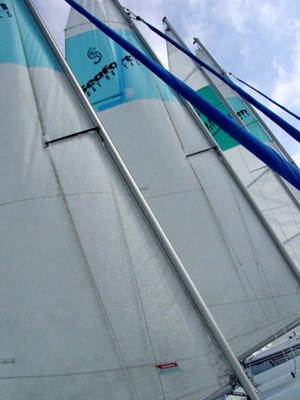The image captures four sailboats lined up next to each other, viewed predominantly from the sails upward. Each sail is primarily white and features a distinct color scheme at the top, with the first sail adorned in teal mixed with black lettering and the subsequent sails displaying variations of teal and deeper greenish colors, each marked with a capital letter 'S' followed by some unreadable writing. Taut ropes and straps, essential for maneuvering the sails, are clearly visible, descending from the masts. The masts themselves, mostly chrome on the first boat and royal blue on the others, pierce through a partially cloudy sky. The decks of the boats, though mostly obscured, appear to be white. A dark blue, unused front sail is wrapped up, adding a touch of contrast to the otherwise uniform scene. The image, taken outdoors with a regular camera, emphasizes the intricate details of the sails and rigging against the backdrop of a light blue sky with white clouds.